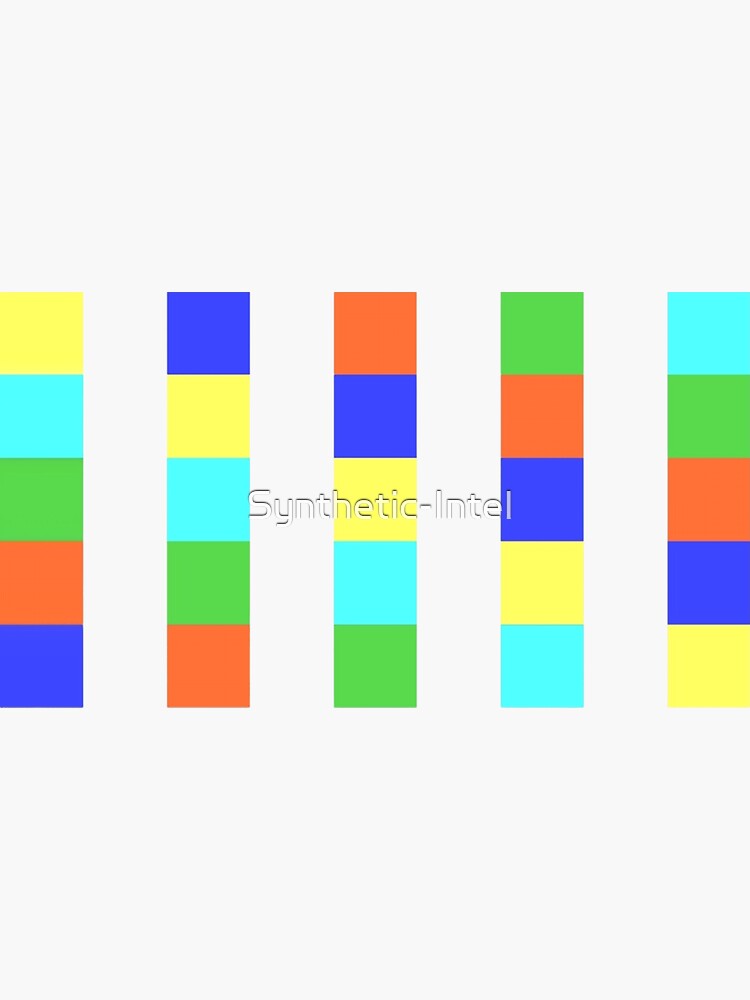The image features a portrait-oriented layout with five vertically aligned rectangles, each made up of five colorful squares. The columns consist of alternating colors in a specific diagonal pattern. Starting from left to right, the sequence of colors in the first column is yellow, cyan (aqua), green, orange, and blue. The second column rearranges these colors, starting with blue at the top, followed by yellow, cyan, green, and orange. The third column begins with orange, then blue, yellow, cyan, and green. In the fourth column, green leads, followed by orange, blue, yellow, and cyan. The fifth column starts with cyan and continues with green, orange, blue, and yellow. This alternating pattern causes the same colors to line up diagonally across the image. The background is off-white, which contrasts with the vibrant colored squares. At the center of the image, a watermark reads "Synthetic-Intel" in white text, though it is unclear whether it refers to the computer processor company or a form of intelligence or information gathering. The image is devoid of additional context, appearing as an abstract design without an explicit explanation of its meaning or purpose.